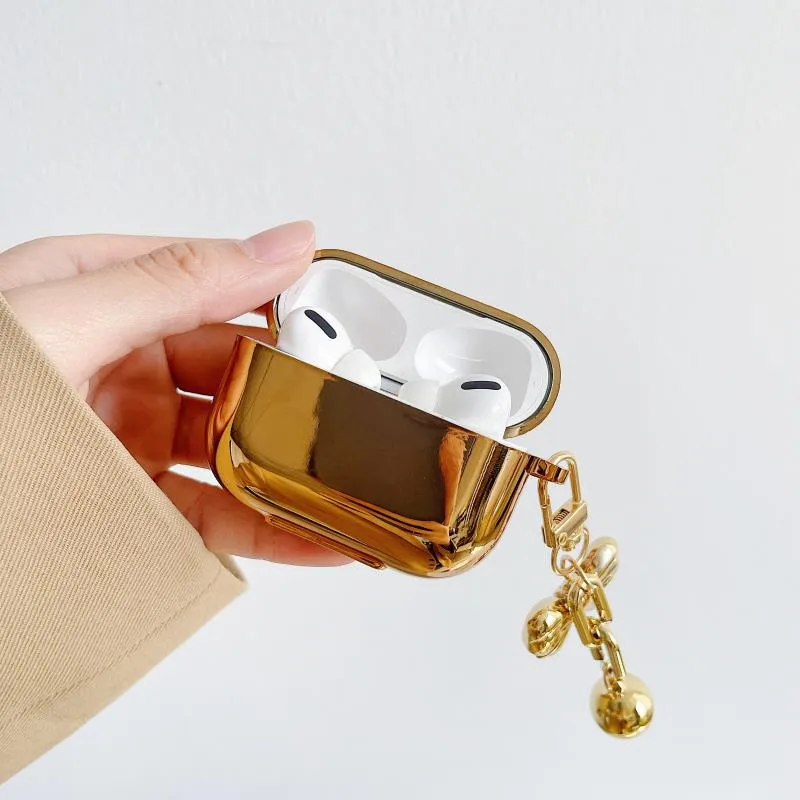In the image, a woman's hand, adorned with long nails and white skin, is delicately holding an open gold AirPods case. The case is shiny and oval-shaped, emitting a reflective gleam. Dangling from the right side of the case is a gold chain with a little ball at the end, designed for attachment purposes. The white AirPods, nestled inside the open case, reveal their black speaker slits. The woman is wearing a textured, khaki-colored, long-sleeve jacket that appears to be made of denim-like material. She grips the case firmly with her fingers and thumb, while her sleeve covers part of her palm. The gray-white background is seamless, showcasing no shadows or shading, with a subtle gradient from a lighter white at the top to a very light gray at the bottom right.